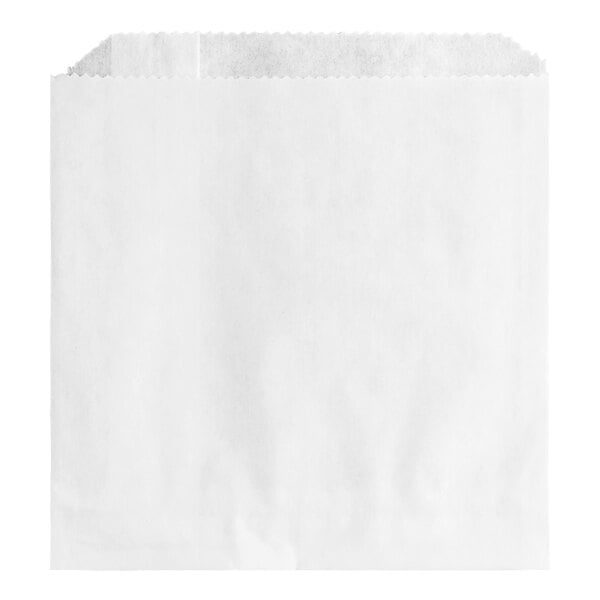This image depicts a small, white paper bag with a corrugated top edge. Captured from a front and slightly elevated angle, the photograph reveals both the front and a glimpse inside the bag, giving a clear view of its rectangular shape. The top of the bag showcases a scalloped, wavy edge across both the front and back. The background is uniformly white, suggesting it may have been edited or taken in front of a white backdrop. The bag's compact size hints at uses such as holding small items like candy bars or greeting cards, reminiscent of bags from a pharmacy or a specialty store.